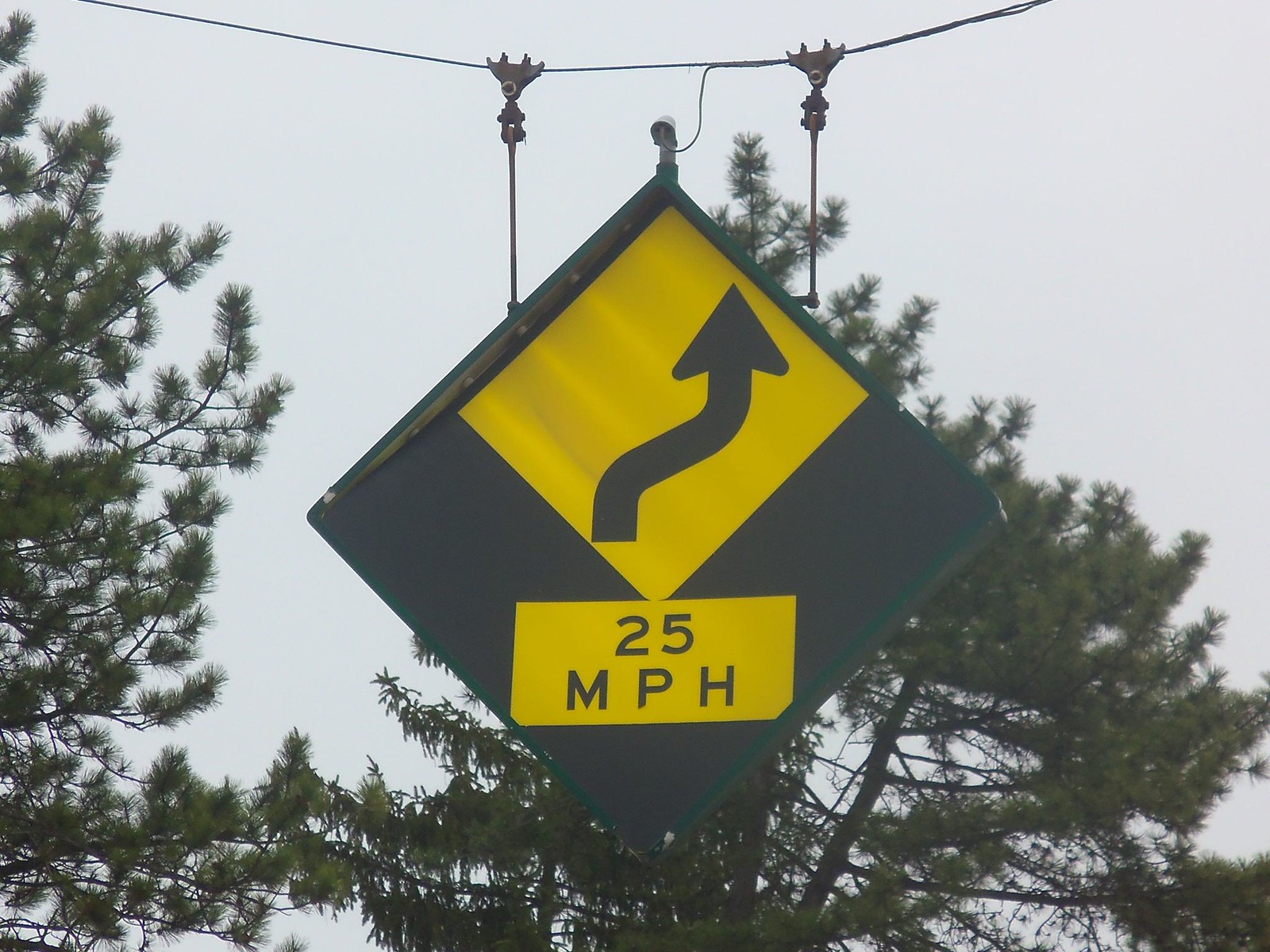This color photograph captures an outdoor scene viewed slightly from below, focusing on a traffic sign suspended from a wire that stretches across what appears to be a street. In the background, you can see leafy trees, and the sky looks overcast, appearing a stark white. The wire spans horizontally across the image, from which a small mechanism resembling claw-like hands is used to hang the sign. The sign is diamond-shaped with a distinctive design: a smaller, yellow diamond nested within, and a bold black arrow pointing upward at the top. Below this nested diamond, there's a yellow rectangular section with "25 miles per hour" inscribed in black, indicating the speed limit.